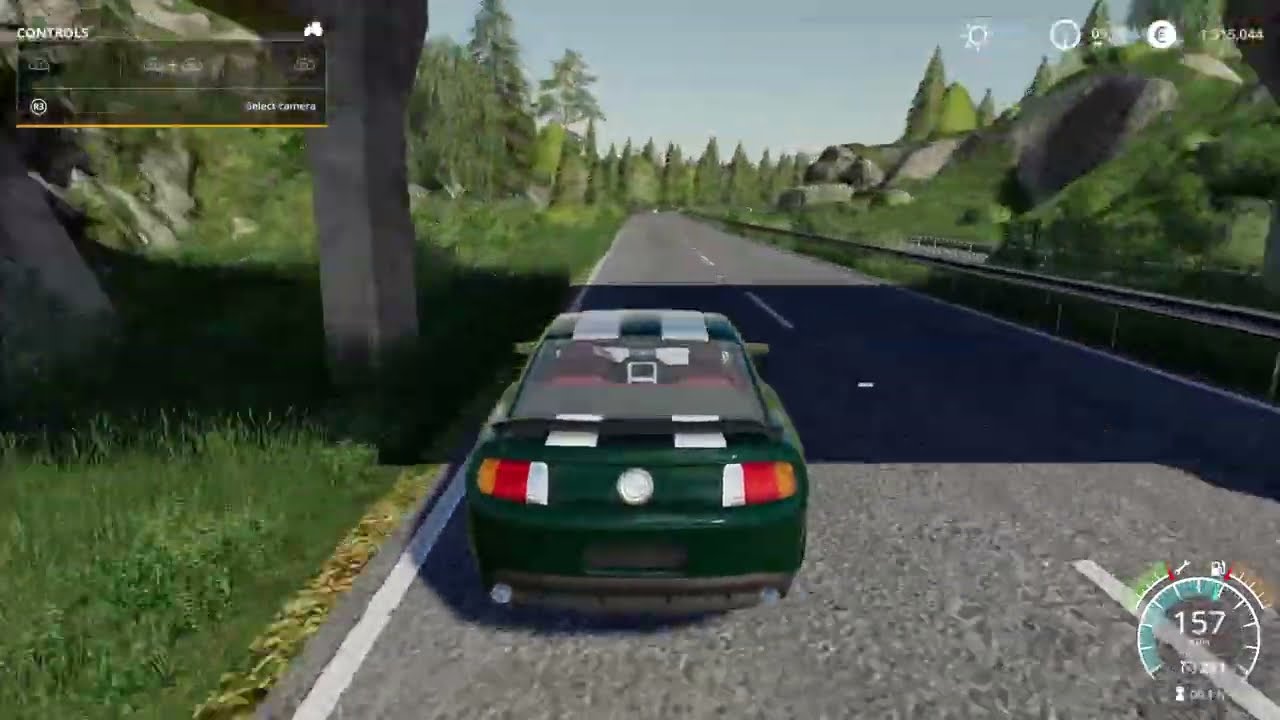The image is a screenshot from a driving video game, featuring what appears to be a new model Ford Mustang. The car is a striking green color with two white racing stripes running down its center. Positioned in the middle of the screen, the Mustang is shown from the rear, revealing a detailed rear fender. The road it is on is a two-lane concrete highway, lined with dashed white lines in the center and solid white lines on either side. The car is traveling at 157 miles per hour, as indicated by the speedometer located in the bottom right-hand corner of the screen. This area also displays gauges for fuel and possible mechanical status.

The highway runs through a lush, green forest, rich with pine trees and other greenery. To the left, the terrain elevates into a mountainous area with grass, bushes, and some gray rocks. To the right, there's a silver guardrail with boulders and mountains beyond it. Additionally, the scene includes a shadow from an overpass above, suggesting the car is driving under a bridge supported by concrete posts.

The game's interface is cluttered with various elements: a control screen in the top left labeled "controls" and referencing a camera, a square area across the top with additional information, including a sunshine icon and other indicators that likely represent the game score. This visually immersive environment aims to mimic an outdoor setting, blending a realistic driving experience with the fantastical elements of video gaming.